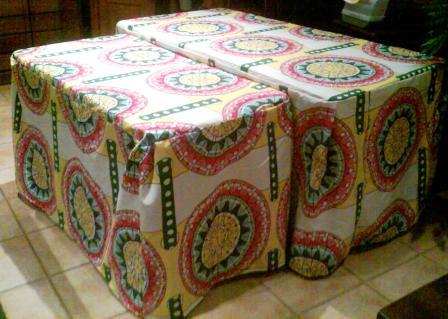This horizontal, rectangular color photograph captures two tables covered with bright, elaborate, floor-length tablecloths featuring intricate designs. The tables are positioned on a beige tiled floor with a small piece of wood, possibly a chair or table leg, in the lower right-hand corner. The tablecloths are adorned with large, circular motifs that resemble suns, characterized by yellow centers and green rays, encircled by red and sometimes blue and green outer rings. These sun-like designs are set against alternating wide yellow and white stripes. Green bars with white polka dots run between the circular patterns, adding another layer of complexity. In the background, there is a brown wooden wall, a square green object in the upper right corner, and possibly a hint of fake plant leaves at the very edge. There are no textual elements on the tablecloths. The vivid, colorful designs evoke a vibrant, festive atmosphere, reminiscent of Mexican or Indian cultural patterns.